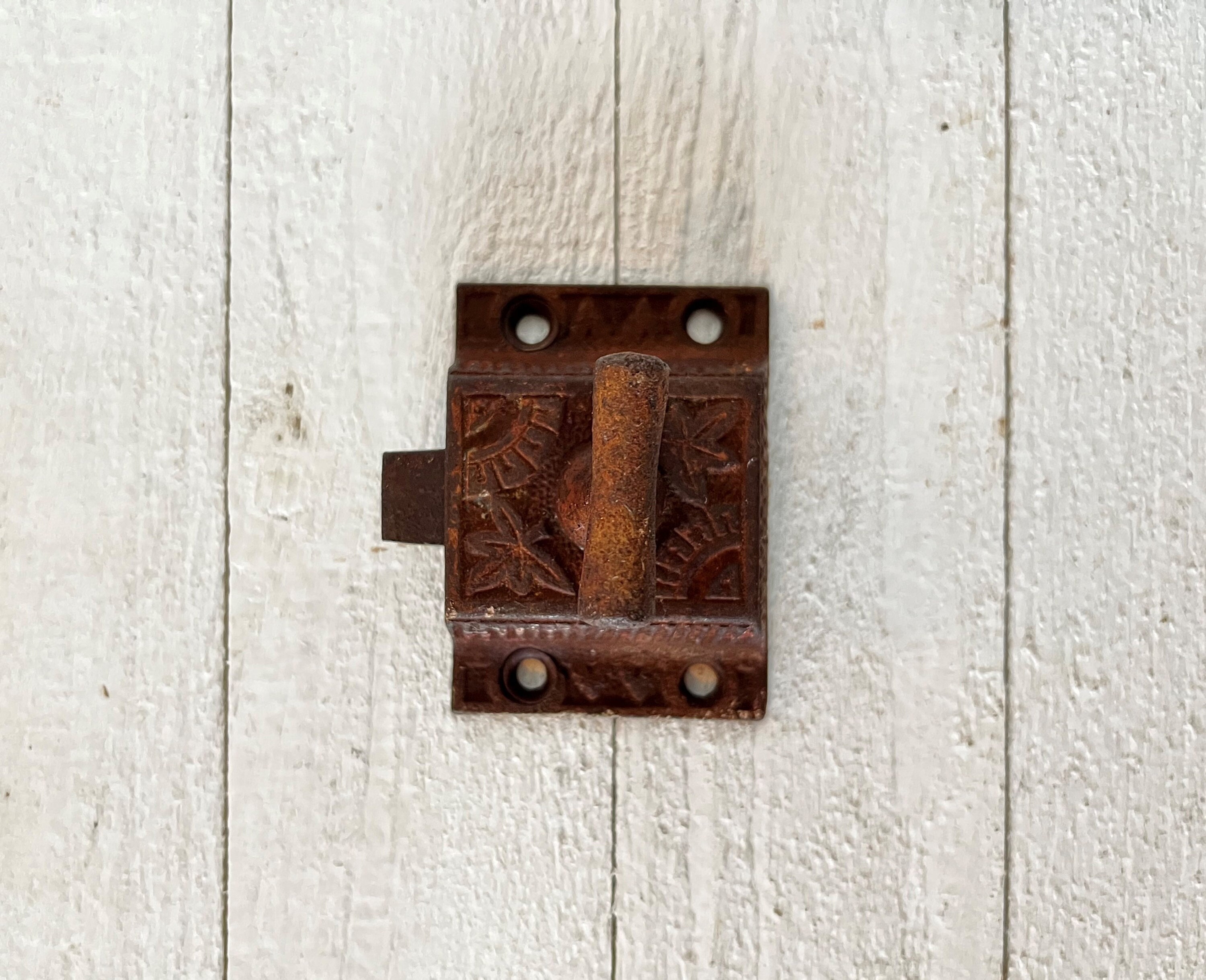The image captures a square, full-color photograph taken outdoors, showcasing a distinctly textured background of white-painted wooden panels, separated by visible black vertical lines. At the center, there is an old, heavily rusted mechanical clasp, displaying a rich, brownish-orange patina. The rectangular clasp features two screw holes at both the top and bottom, and it is adorned with intricate geometrical and leaf designs within its body. The top of the clasp sports a rusty handle or lever that seems functional. On the left side of the device, there is a component that looks like part of a locking mechanism, suggesting it could be used to secure something. The absence of any screws implies the clasp is merely resting against the white wood panels rather than being fixed in place, lending a further air of antiquity and disuse to the scene.